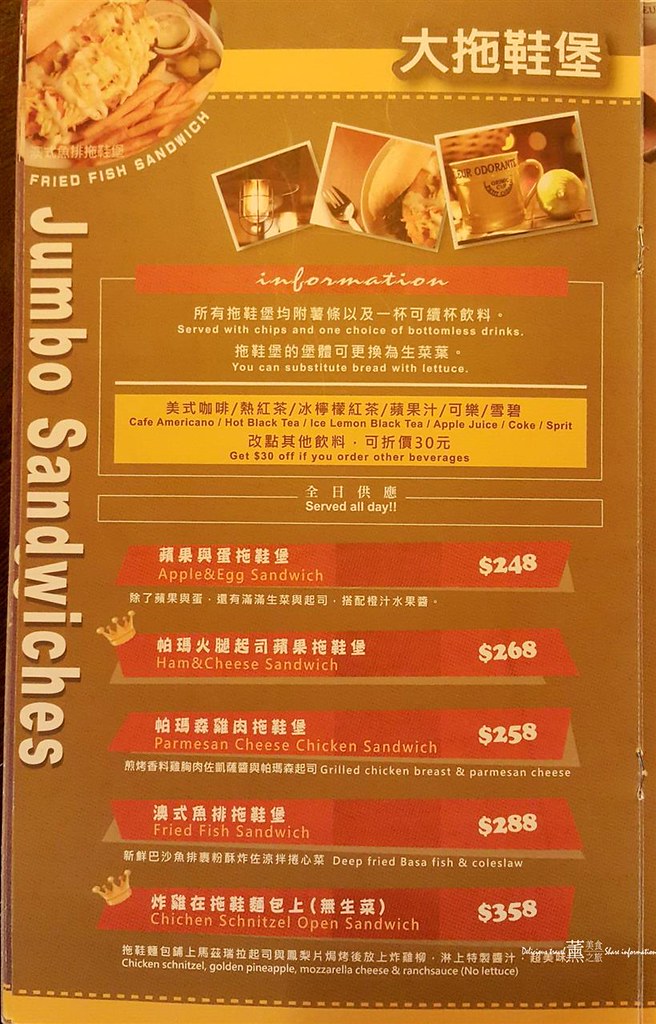A detailed caption for the image might read:

"The image displays a restaurant menu featuring Asian characters prominently in a large size at the top right. These characters, which appear to be the restaurant's name, are white with a brown outline. At the top left, the menu highlights a featured dish, showcasing a tempting fried fish sandwich with a side of fries, onions, and pickles, all depicted in a vibrant photograph. The overall menu has a brown background, creating a warm and inviting aesthetic. Along the left side, the phrase 'Jumbo Sandwiches' is presented vertically in bold white text. A section towards the top features a yellow background with 'Beverages' listed in both Asian characters and English, indicating a variety of drink options. Below this, different sandwich offerings are categorized within a section marked by a red background, creating a visually engaging and easy-to-navigate menu layout."